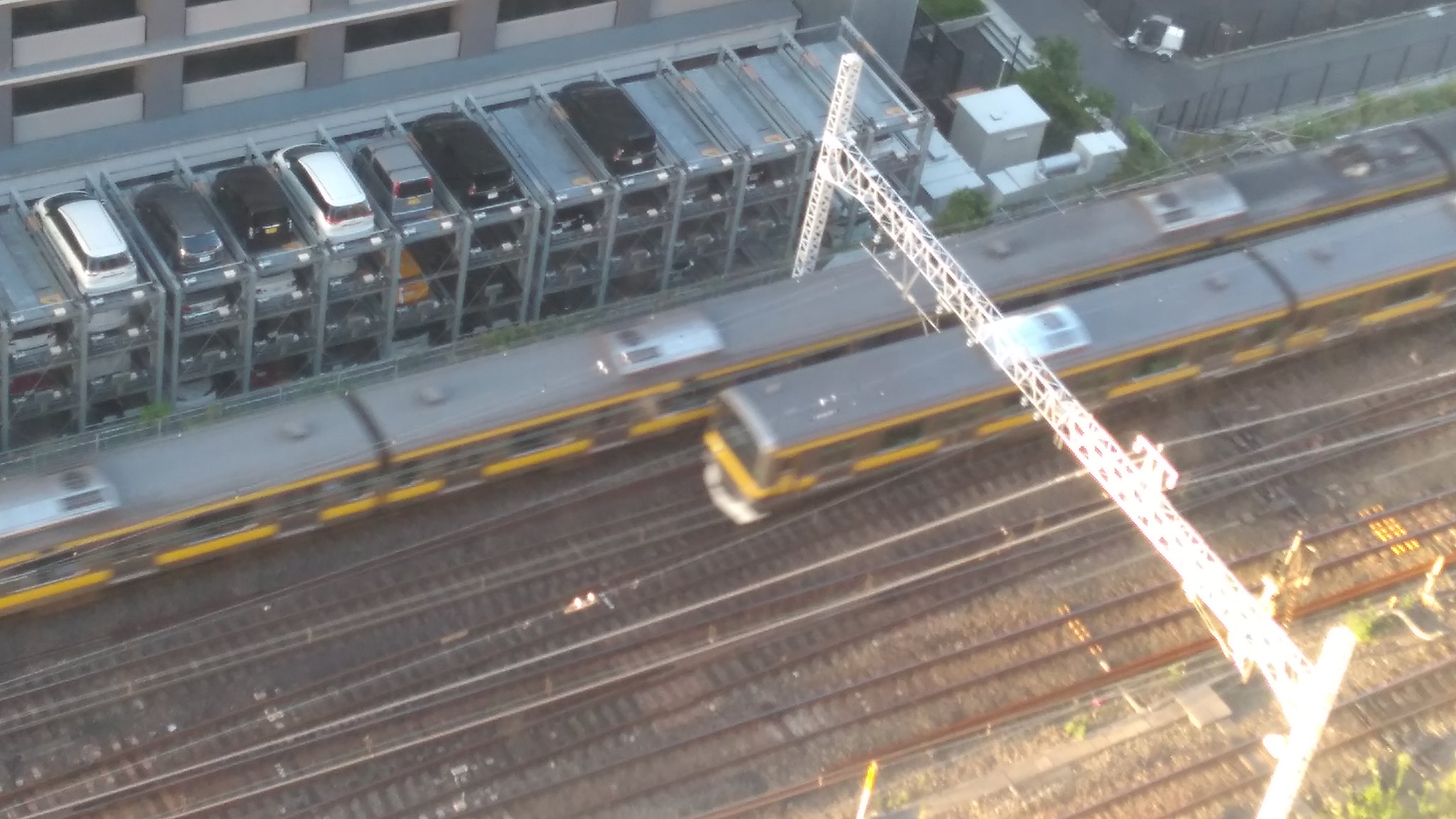This vibrant color photograph provides an aerial view, captured from approximately eight or nine stories high. It depicts a scene of multiple train tracks—about five or six—cutting through the frame diagonally, with two yellow and grey commuter trains visibly in motion, their slight blurriness accentuating their speed. Near the top left corner of the image, a parking garage stands prominently, its grey metal structure offering a striking contrast to the scene. This garage houses a number of cars, including a white, brown, black, and silver one among others, arranged meticulously within their cubical spaces. The area surrounding the train tracks includes smaller white buildings and a greyish concrete parking lot or road. Under the bright sunny sky, which washes out part of the photo with its brilliance, a white metal structure crosses the tracks towards the right of the image, adding an intriguing architectural element to the dynamic urban landscape.